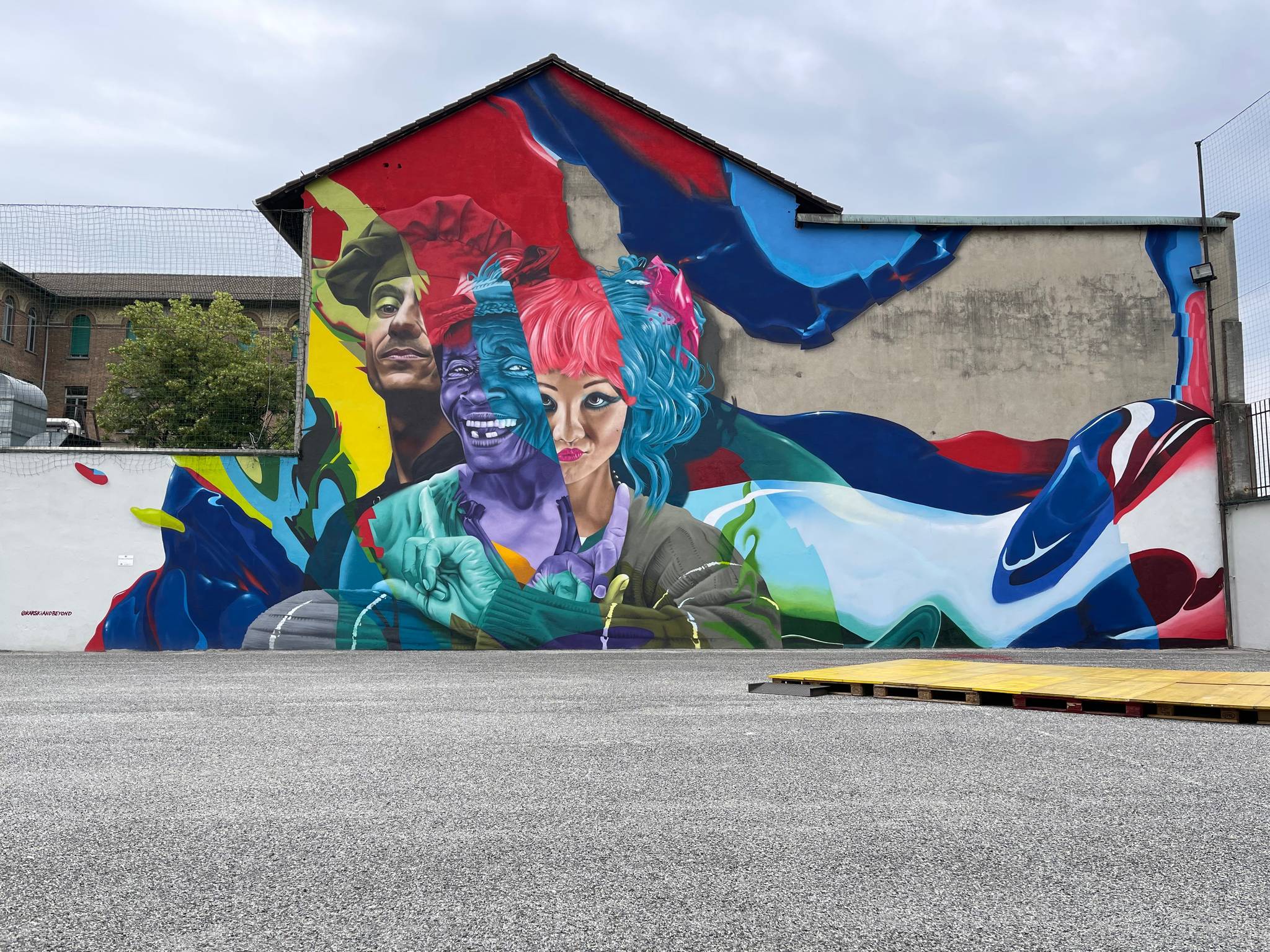The image showcases a vibrant and detailed mural painted on the side of a concrete building. This art piece features three distinct figures: on the left, a white man wearing a chef's hat; in the middle, a smiling man donning a paperboy hat; and on the right, an Asian woman with striking pink and blue hair. The background of the mural is an abstract swirl of red, white, and blue, adding to its dynamic composition. The unpainted section of the building reveals a peaked roof at the center and a flat roof on the right, tapering down to the left. The surrounding area includes black asphalt in the foreground, a large line of wooden pallets on the right, and to the left, the visible brick wall of a nearby house and a protective fence. Beyond the wall, a courtyard with a tree can be seen, adding a touch of natural greenery to the urban setting. A yellow plywood pallet lies on the ground, adding a splash of color to the scene.